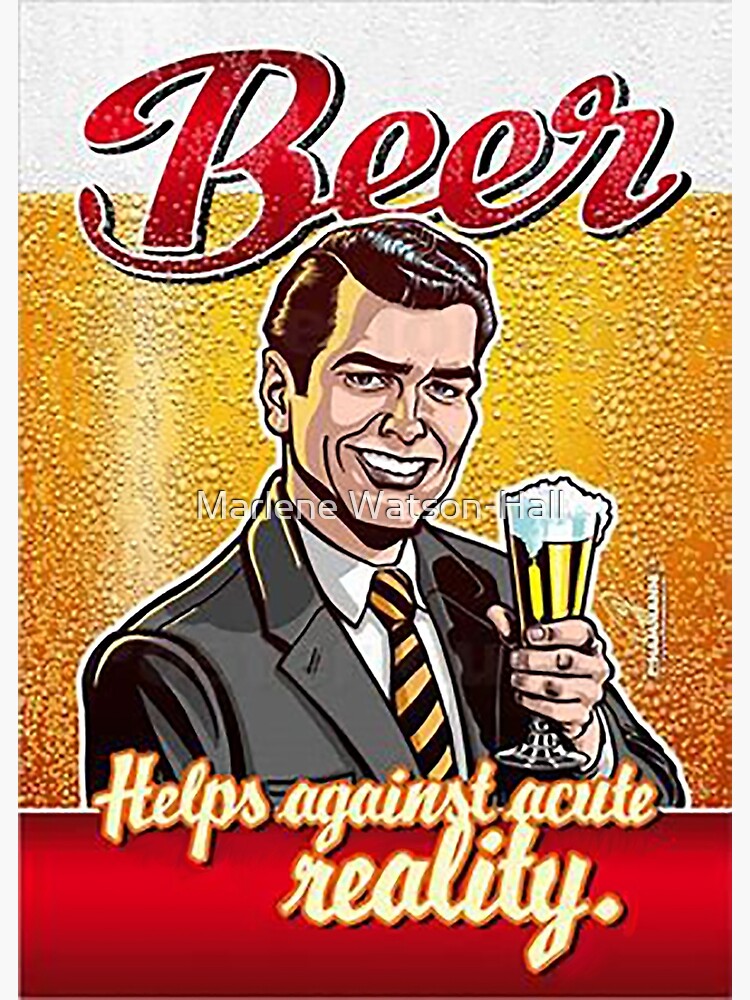The image is an old-timey, comic-style advertisement for beer. At the top, a red cursive script spells out "beer" over a white background that resembles the foam on top of a freshly poured beer. Below the foam, the background consists of a bubbly golden-yellow liquid, simulating the appearance of beer in a glass bottle or a tall glass. The bottom 20% of the poster is red and features the phrase "helps against acute reality" in yellow text.

In the center of the image is an illustration of a man with brown hair, neatly parted on the side. He is smiling and dressed conservatively in a grey suit jacket over a white button-up shirt and a striking black and yellow striped tie. In his left hand, he proudly holds up a tall glass of beer with a generous amount of white foam spilling over the top. There is a watermark on the image that says "Marlene Watson Hall." The overall effect is vintage and comedic, capturing both the visual and textual elements of early beer advertisements.